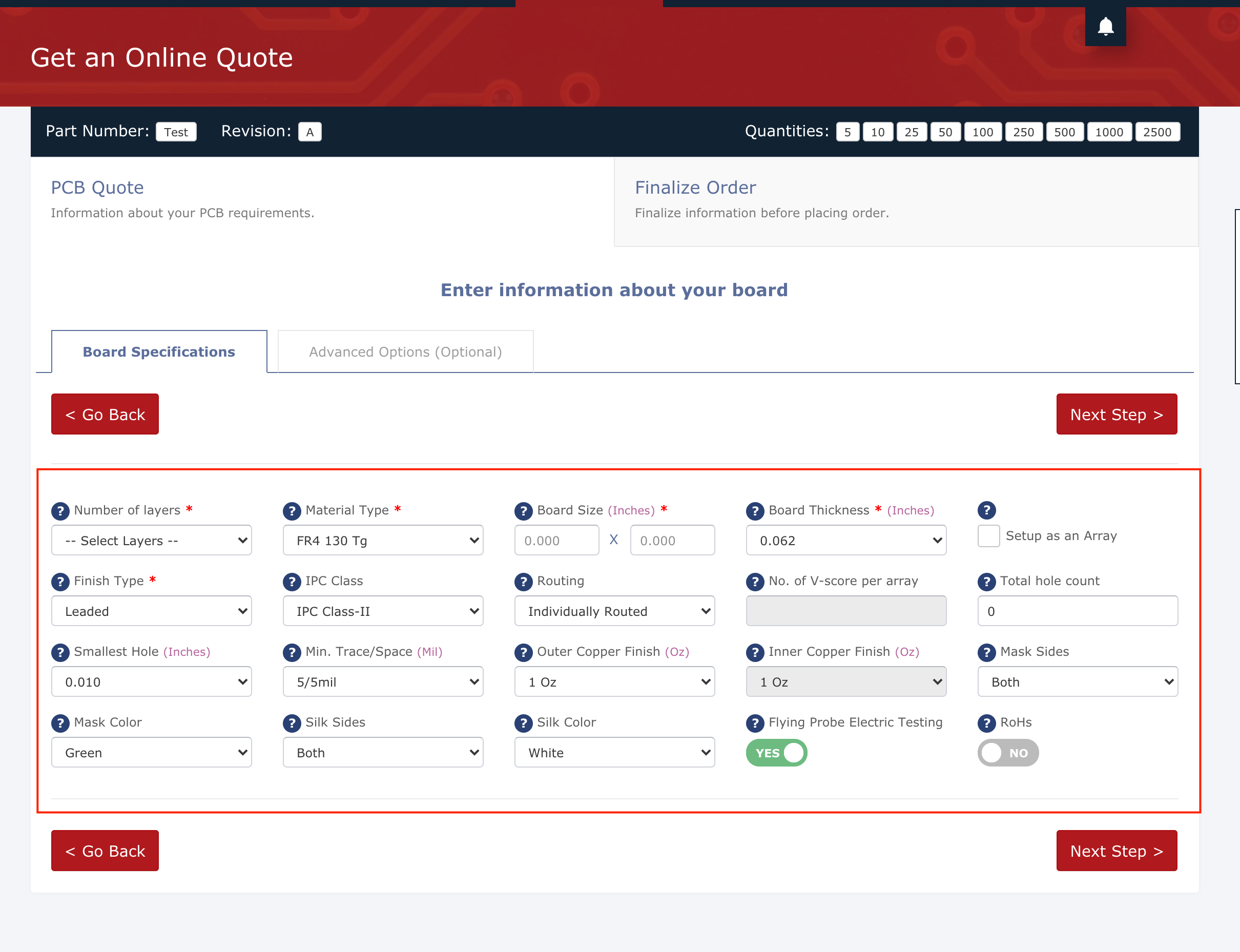In the upper left corner of the image, a red strip hosts a white text box with the words "Get a Quote, Get an Online Quote." To the right, a white bell icon for notifications is set against a small blue square. Below the banner, a black strip has various labels; on the left, it features a white button labeled "Part Number Test" with the text "Test" in black, followed by another white button labeled "Revision" featuring the letter "A."

On the right side of this strip, the term "Quantities" is spelled out in black font, with a series of white buttons displaying different numbers: 5, 10, 25, 50, 100, 250, 500, 1000, and 2500. Further down, on a white background, the heading "PCB Quote" appears, along with information about your PCB requirements. To the right, there are instructions to "Finalize Order" and "Finalize Information Before Placing Order."

Centered in the middle below this section, the text "Enter Information About Your Board" is displayed above two tabs: "Board Specific Specifications" and "Advanced Options (Optional)." "Board Specific" is in blue font, while "Specifications" is in gray, both set against a white background. Below these tabs, a red button with white font reads "Go Back," and another red button with white font on the right says "Next Step."

Beneath these buttons, a detailed chart is outlined in red, presenting an array of options. From the left, it cites "Number of Layers" with a dropdown menu to select the number of layers. "Finish Type" also features a dropdown menu, with "Leaded" being one of the options. "Smallest Hole (inches): 0.010" appears next, followed by dropdowns for "Mask Color" (green) and "Material Type" (FR4 130 TG). The term "ICE" follows at the end of this detailed list.